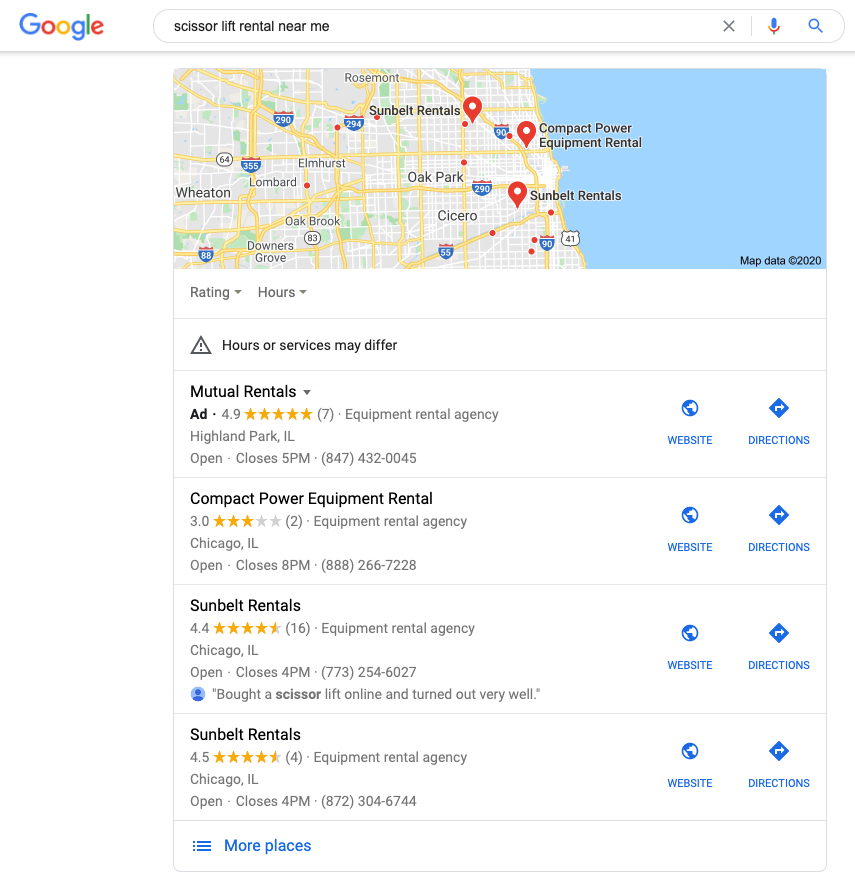The image displays a computer or tablet screen featuring a Google search page. The iconic Google logo appears with "G" in blue, "o" in red, "o" in yellow, "g" in blue, "l" in green, and "e" in red. The search bar contains the query "scissor lift rental near me," accompanied by a gray "X," a line, a microphone icon, and a blue magnifying glass icon.

Below the search bar is a detailed map highlighting several locations including Oak Park, Elmhurst, Oakbrook, Downers Grove, Wheaton, and Cicero. Markers on the map identify nearby companies offering scissor lift rentals: Compact Power Equipment Rental, and two branches of Sunbelt Rentals.

Beneath the map, there are options to filter or sort results with dropdown menus labeled "Rating" and "Hours," both indicated by downward-pointing triangles. An alert icon with an exclamation mark cautions: "Hours or services may differ."

The search results detailed below include:

1. **Mutual Rentals (Ad, 4.9 stars with 7 reviews)**
   - Location: Highland Park, Illinois
   - Status: Open, closes at 5 PM
   - Contact: 847-432-0045

2. **Compact Power Equipment Rental (3 stars, 2 reviews)**
   - Location: Chicago, Illinois
   - Status: Open, closes at 8 PM
   - Contact: 888-266-7228

3. **Sunbelt Rentals (4.4 stars with 16 reviews)**
   - Location: Chicago, Illinois
   - Status: Open, closes at 4 PM
   - Contact: 773-254-6027
   - User Testimonial: "I bought a scissor lift online and turned out very well."

4. **Sunbelt Rentals (4.5 stars with 4 reviews)**
   - Location: Chicago, Illinois
   - Status: Open, closes at 4 PM
   - Contact: 872-304-6744

Each listing features icons for "Website" (globe icon) and "Directions" (diamond with right arrow icon).

At the bottom, a button labeled "More places" appears in blue, represented by three bullet points with three lines next to each.